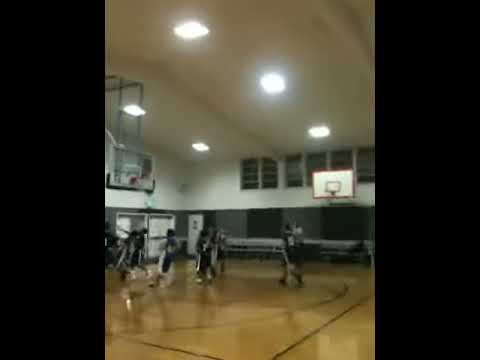The photograph captures an indoor high school gymnasium, likely used for sporting events. The gym has a high ceiling with suspended overhead lighting that brightly illuminates the scene. The floor is a polished brown wood, marked with clear basketball court lines. The gymnasium's lower walls are dark grey, transitioning to white at the upper levels, and feature doorways and openings. Overhead, there’s a balcony with windows. 

In the middle of the court, about seven players in black and white uniforms are engaged in activity. Some are running, creating a blurred effect, indicating movement and possibly an ongoing game or a practice session. To the left of the photo, a basketball hoop is suspended from the ceiling, while another hoop is on the right side, with its white backboard halfway up the wall. The absence of spectators and the precise formation of the players suggests a practice session or drill, rather than an actual game.